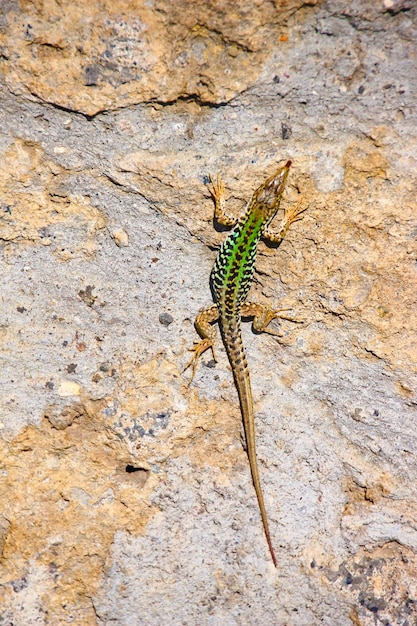The photo captures a small lizard perched on a flat expanse of grayish, tan-speckled rocks. The rocks are flecked with patches of peachy color, and scattered with tiny white and black pebbles, possibly remnants from erosion. The lizard, situated slightly to the right of the image’s center, is a darker tan than most of the rocks, and is gazing off to the right. His body displays a checkerboard pattern of black and white specks along the sides, while bright fluorescent green highlights run parallel to his spine. His pointed snout and four feet, each with long toes and tiny claws, highlight his detailed form. The lizard's head, tail, and feet are a peachy tan, contrasting with the brown stripe running down his otherwise green body. Despite the intricate details, the lizard occupies only a small portion of the photograph, resembling a delicate, linear figure against the rock's broad surface.